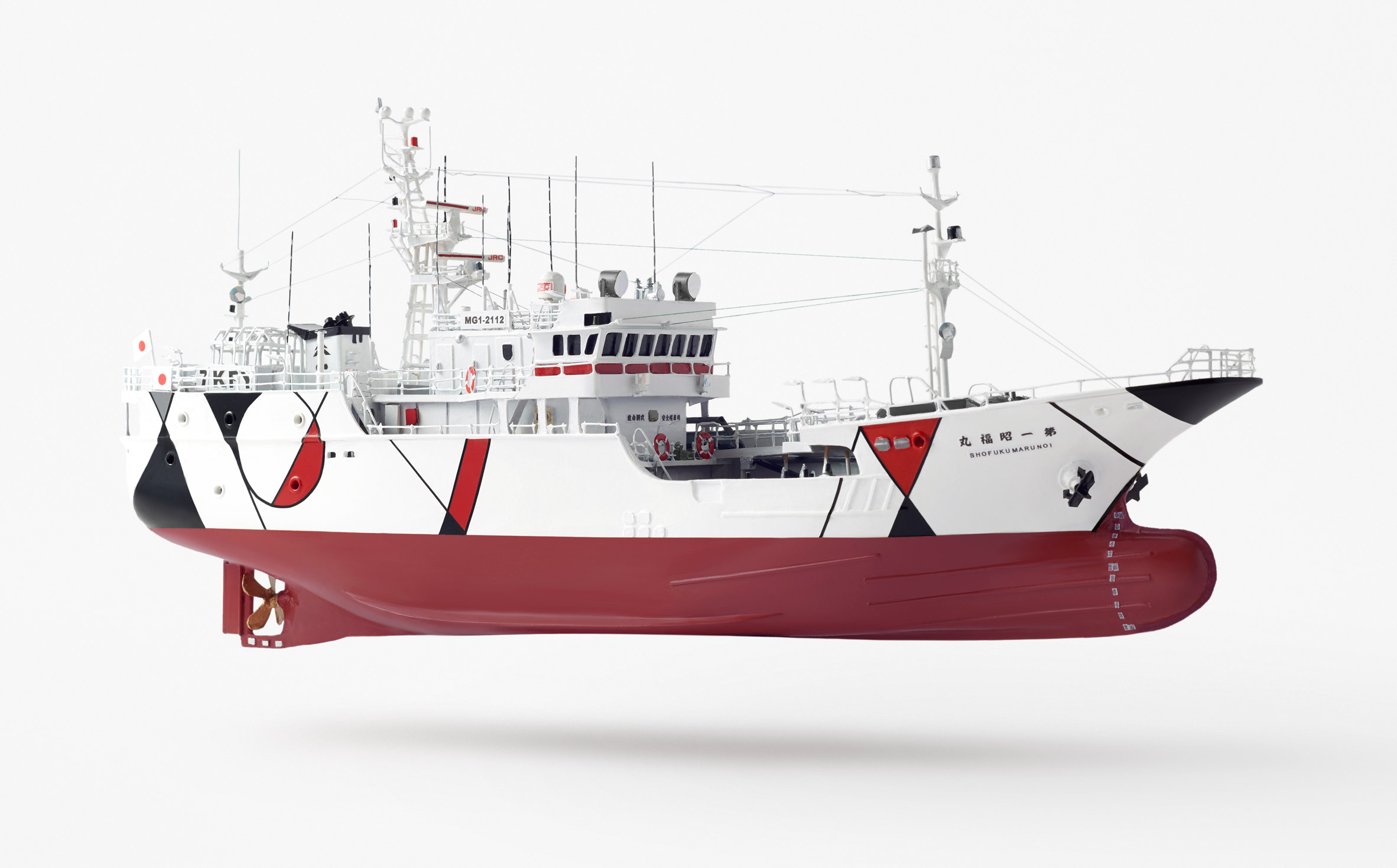This photograph showcases a highly detailed miniature model of an ocean vessel, floating a few inches above a dark white background. The hull, painted a striking reddish-brown, transitions to white above the waterline where red and black geometric patterns, including triangles and circles, embellish the sides. Notably, blue shapes and what seem to be Asian characters are also present, hinting at the vessel's identity. The model features three prominent towers and numerous slender antennas in its midsection. The central control tower has multiple darkened windows, adding to the realistic appearance. Additional details include visible propellers at the stern, white safety barriers along the deck, and connecting lines and cables that enhance the ship's intricate design. The overall meticulous craftsmanship captures both the vessel's structure and its intricate deck layouts, complete with lights and other maritime features.